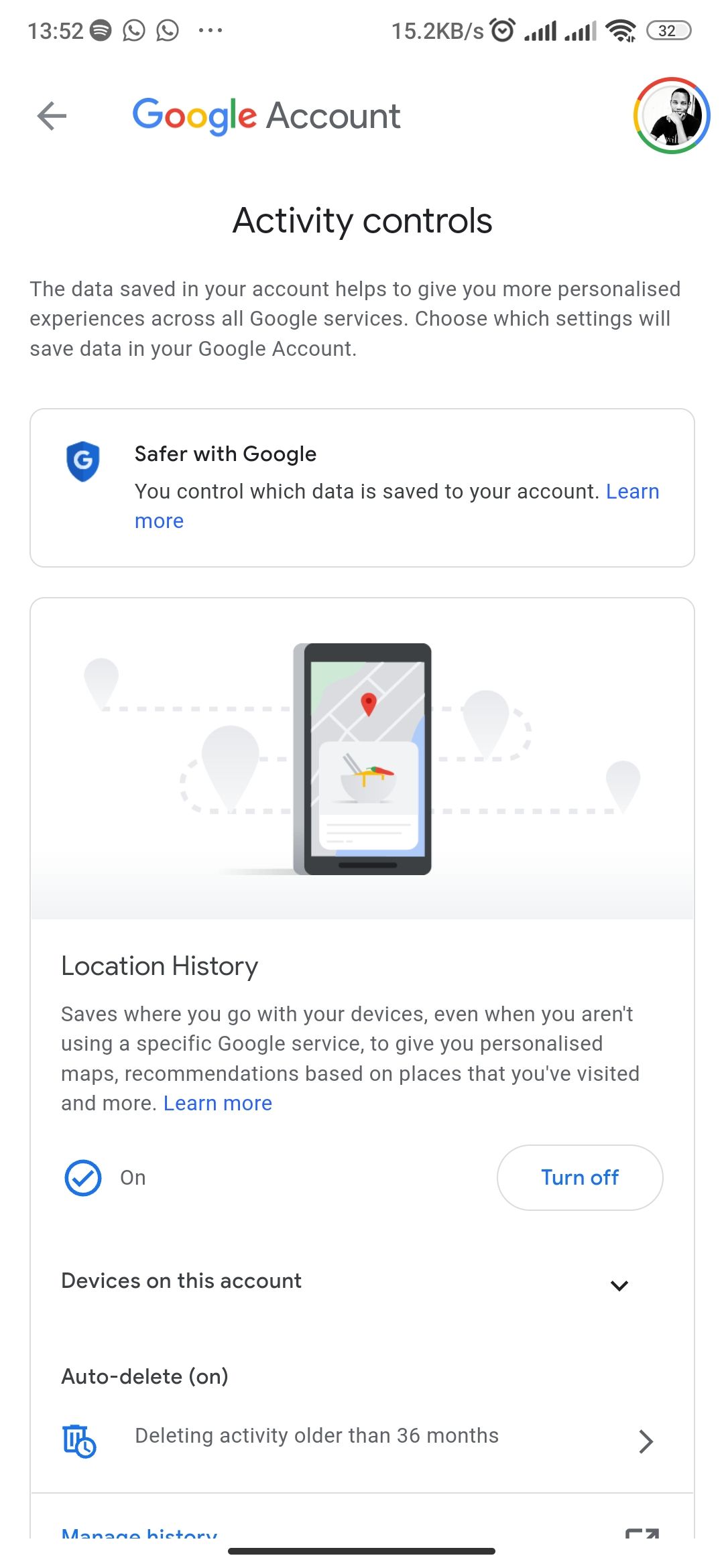This screenshot, taken from the Google Account website, depicts the Activity Controls settings screen, focusing on accessibility options. The user navigates through these settings, displaying a sense of skepticism toward Google’s data handling practices. In the upper right corner, a profile picture associated with the Google Account is visible. Currently, the user has Location History enabled, but they might be considering disabling it after scrutinizing the settings. A prompt from Google assures users of enhanced safety and greater control over their data, a claim open to personal interpretation. Additionally, there is an option for auto-deleting activity data after 36 months, offering users a measure of privacy management.